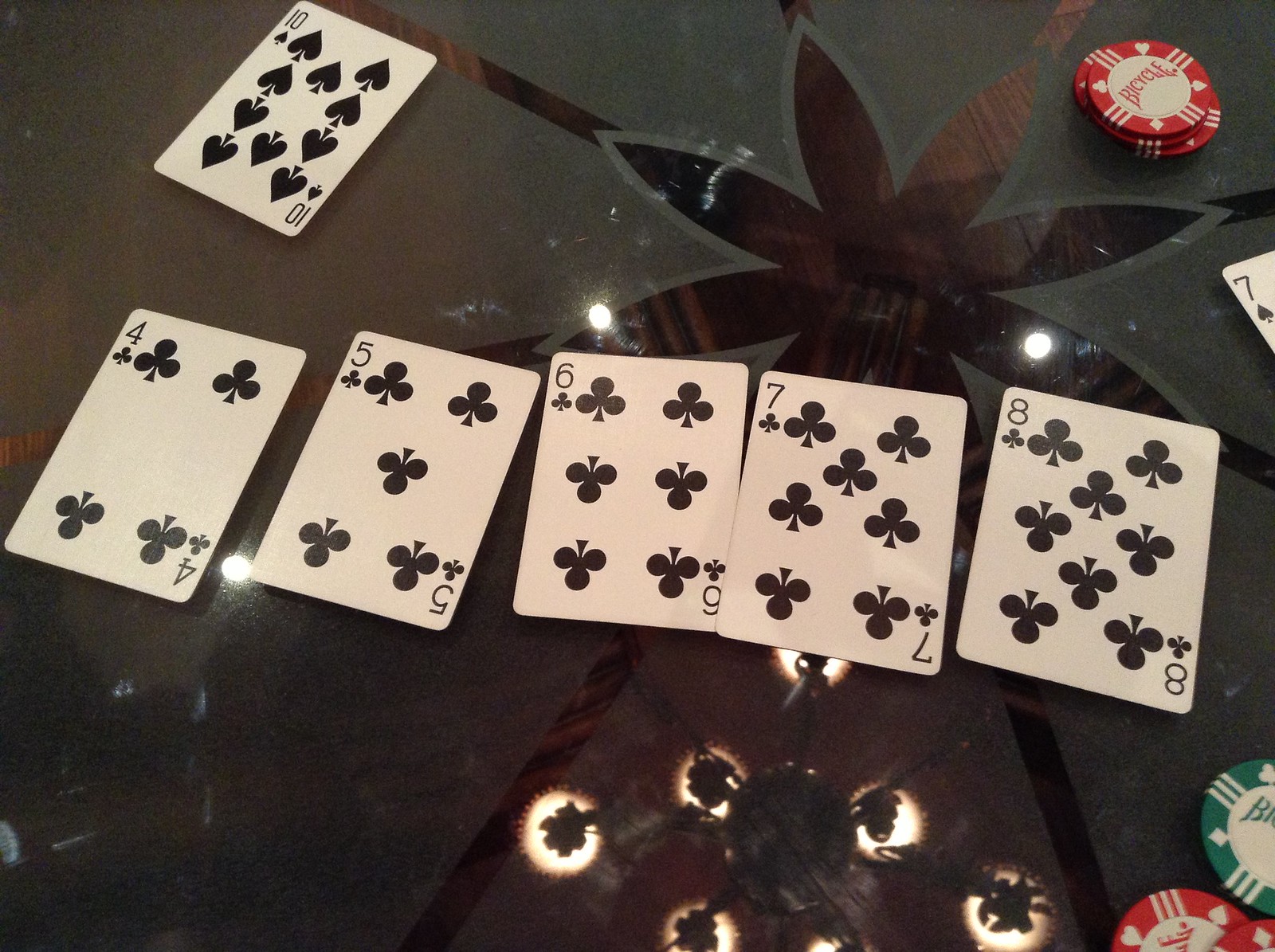A top-down photograph captures an intense game of Texas Hold'em on a glass table, adorned with a frosted floral design. The community cards laid out are the four through eight of clubs, accompanied by the ten and seven of spades. Among the stakes are red and green Bicycle chips, indicating significant bets. The glass table reflects an old-fashioned chandelier hanging overhead, adding a touch of elegance to the scene. Additional overhead lights are also visible in the reflection. Below the table, a dark wood floor provides a rich contrast to the game's vibrant elements, completing the atmospheric setup.